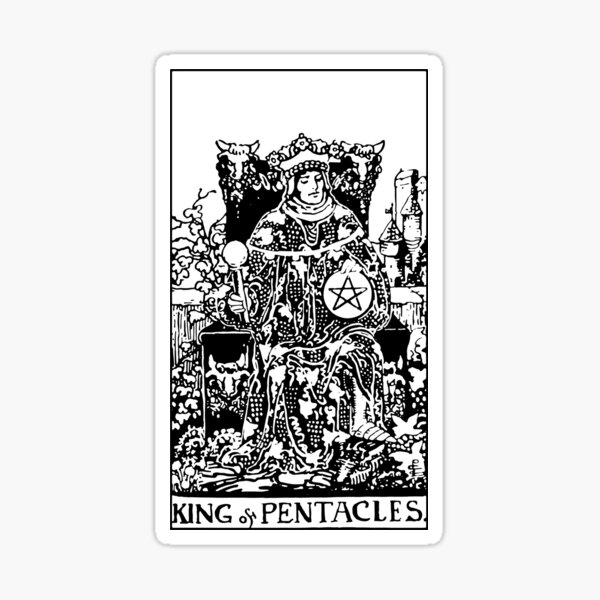This black and white image depicts a tarot card labeled "King of Pentacles." At the center is an ornate depiction of a king seated majestically on a richly adorned throne. In his left hand, he holds a scepter aloft, while his right hand rests on a pentacle—a circular object featuring a five-pointed star with the top point oriented upwards. The king is garbed in elaborate robes and wears a crown signifying his authority.

The throne itself is decorated with bull's heads at the top corners and armrests, giving it a distinctive and regal appearance. In the background to the right stands a castle, adding to the grandeur of the scene. Below the king, the illustration becomes intricate and busy, with various plants and ornamental details interwoven into the design. The monochromatic nature of the artwork, rendered without shading, creates a detailed yet stark contrast, enhancing the classical, Renaissance-like style of the illustration. The entire image is framed by a white border, reminiscent of a playing card.